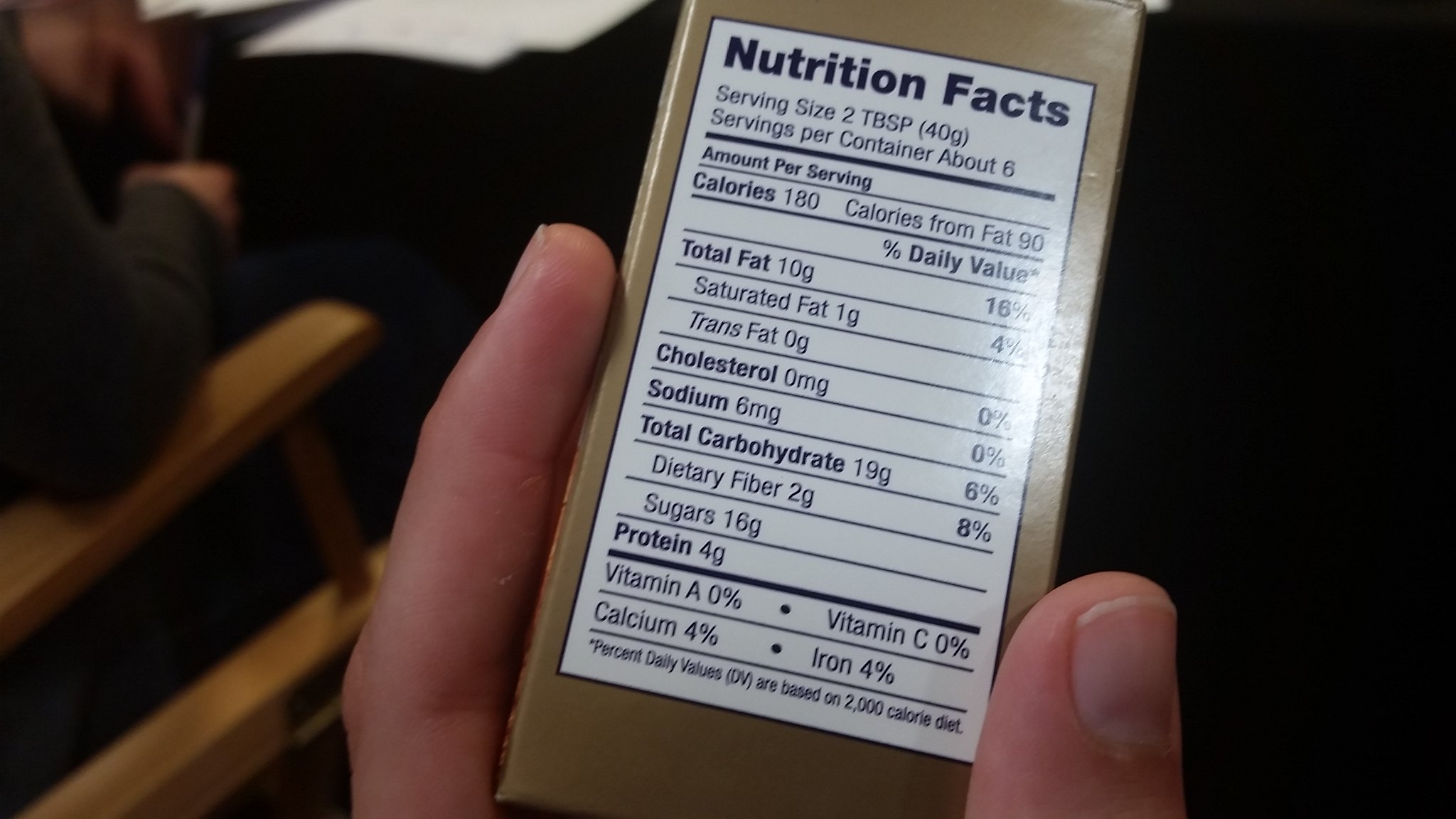In the image displayed on the screen, a hand with short, well-manicured nails is seen gripping a light brown food box. The hand holds the box on its shorter side, where the nutrition facts label is visible. According to the label, a serving size is 2 tablespoons (40 grams), with approximately 6 servings per container. Each serving contributes 180 calories, of which 90 calories are from fat. The nutritional breakdown includes 10 grams of fat (1 gram saturated), no trans fat, no cholesterol, 6 milligrams of sodium, 19 grams of carbohydrates (2 grams dietary fiber, 16 grams sugars), and 4 grams of protein. Additionally, each serving provides 4% of the recommended daily allowance (RDA) for both calcium and iron, based on a 2,000 calorie diet. The image has been taken in a well-lit environment, as evidenced by the light reflection on the right side of the box. The hand, seen from the forefinger and thumb wrapped around the bottom of the box, indicates careful handling.